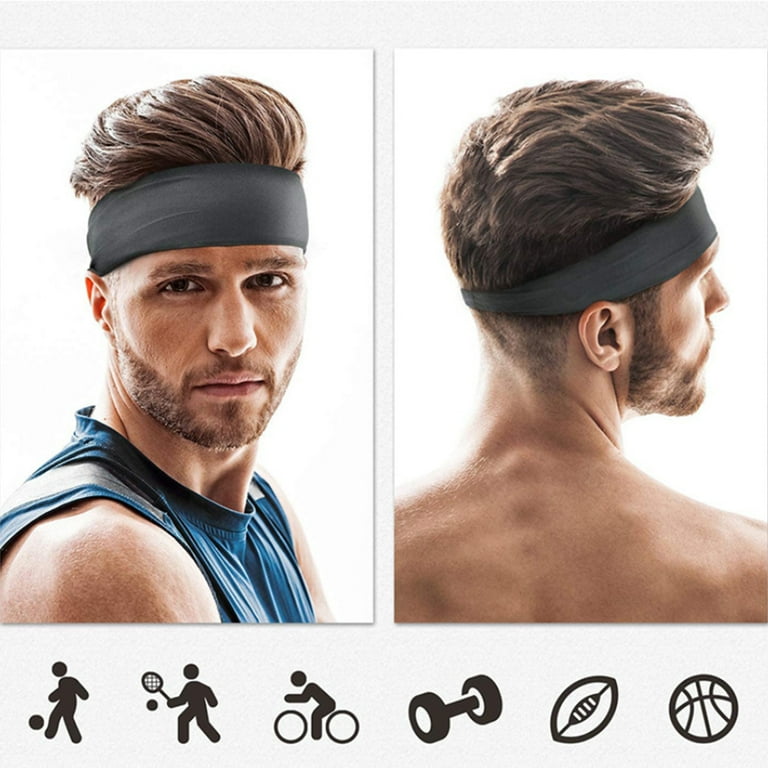In the image, we have a split-screen featuring two pictures of the same man. In the left image, the man is wearing a blue and gray tank top. He has a well-groomed beard and mustache and is Caucasian. His hair is tall, puffy, and brown, slicked back as if styled with a lot of hair gel. He also wears a blackish-gray headband across his forehead. The man is facing sideways but has turned his head to the front, displaying his dark eyes. The right image shows the man from the back, shirtless, revealing the same puffy, layered hair with the bottom part of his head shaved. Despite the different angle, he wears the same headband. The backdrop of the images is a grayish-white, and along the bottom of the screen, there are black stick-figure silhouettes depicting various sports activities: one kicking a ball, one playing tennis or badminton, one riding a bicycle, followed by icons of a dumbbell, a football, and a basketball.